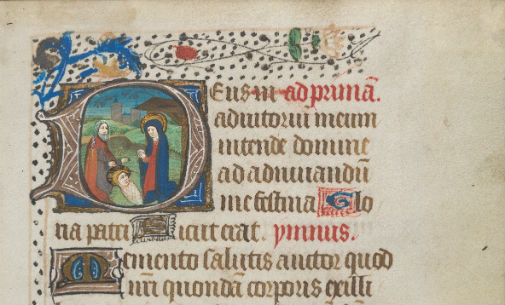This image depicts an ancient, horizontally-aligned rectangular piece of paper with a faded, light brown background, accented by darker stains. The page, which appears to be from an old book, features text and illustrations believed to have significant religious or historical relevance. On the left side of the paper, enclosed within a large, circular ornament resembling a backwards lowercase 'A,' is a detailed image that likely represents a religious scene, possibly of Joseph, Mary, and Baby Jesus, with figures donned in colorful robes. One figure resembles a nun in a blue or red robe, while another character, presumably male, has a gray beard and wears an orange and red robe. The right side of the image displays a series of neatly organized, right-aligned symbols or characters, spread out in five rows of brown text interspersed with occasional red lettering. Below this segment are three additional rows of these symbols, similarly showing sporadic red words among the brown characters. The writing, which might be in Latin, reflects a mix of black and red ink, contributing to the document's historical aura.